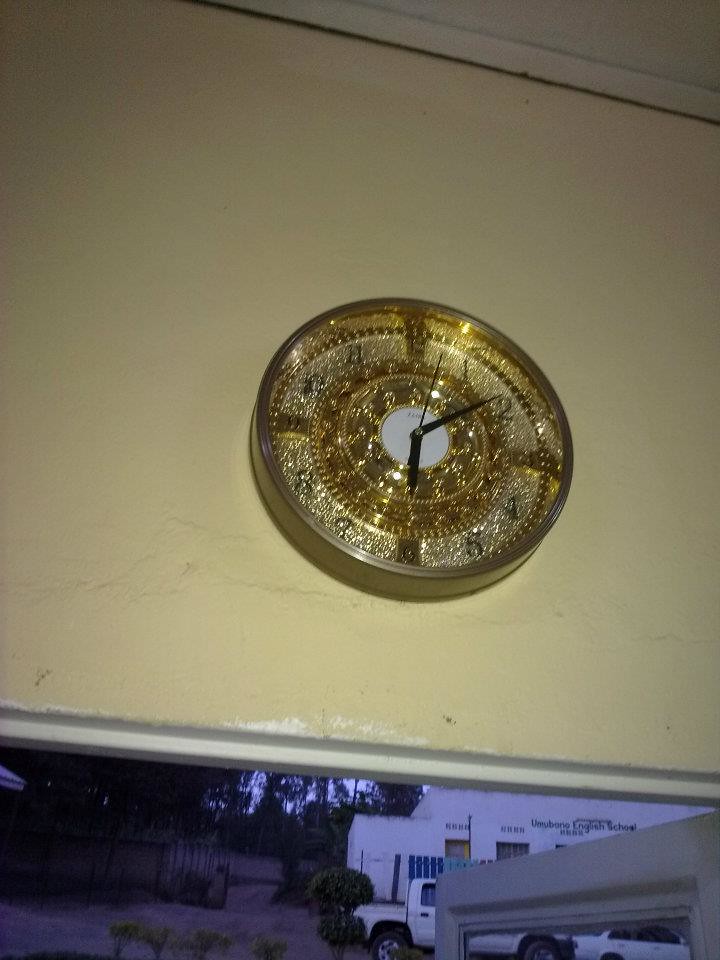The image depicts an ornate, round, golden clock mounted on a wall. The clock features multiple concentric circles with the outermost circle appearing in a dark gold or brass color. Inside these circles, the clock face lightens to a pale gold shade where the numbers are displayed in understated gold lettering. At the center, a stark white circle houses black hour, minute, and thin second hands, displaying a time of approximately 6:09.

The golden clock is affixed to a wall that's primarily yellowish with white trimming along both the top and bottom edges. The upper right corner of the picture peeks into a white ceiling. Below the wall is a window through which one can view a tranquil outdoor scene. This view includes a tree line to the left, and on the right, there is a white building, a white truck, and another white car parked facing right. Additional details outside include a stockade fence, a driveway, and some green bushes, all under a twilight sky. The very bottom right of the picture captures the corner of an open white door with a bit of glass visible.